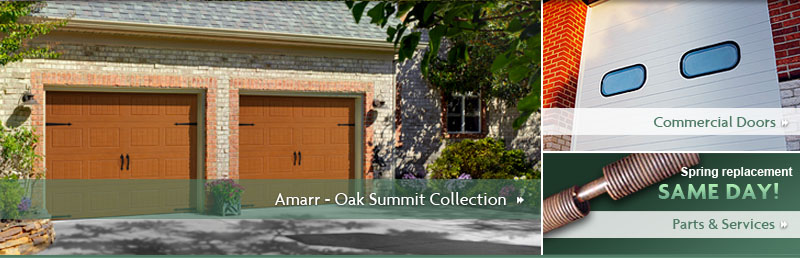This color image showcases a collage of three distinct photos, likely related to commercial property features. 

- **Left Photo:** Depicts a building facade, possibly a garage, with two prominent orangey-brown doors framed by brown, white, and orange brickwork. Above the doors, there's a grey roof, and the scene is flanked by trees on both sides. The ground is covered with grey pavement. A green band near the bottom of the photo bears white text on the right which reads, "Almar Stroke Oak Summit Collection," alongside a small white arrow.

- **Upper Right Photo:** Features a white door adorned with two round blue rectangles. To the left of the door is orangey-red brick, illuminated by sunlight, while the right side displays black and red bricks cast in shadow. Above this image, "Commercial Doors" is inscribed, indicating the nature of the door.

- **Lower Right Photo:** Shows a copper coil with a narrow central section. This image may relate to spring mechanisms used in door systems. The image is topped by a green banner with white text stating "Spring Replacement," followed by a white banner in the center that says "Same Day Parts and Services." At the bottom, another green banner accompanies the image, but only contains a simple design and no text.

Overall, these photos collectively present elements associated with commercial doors, perhaps highlighting the products and services offered for commercial property enhancements.